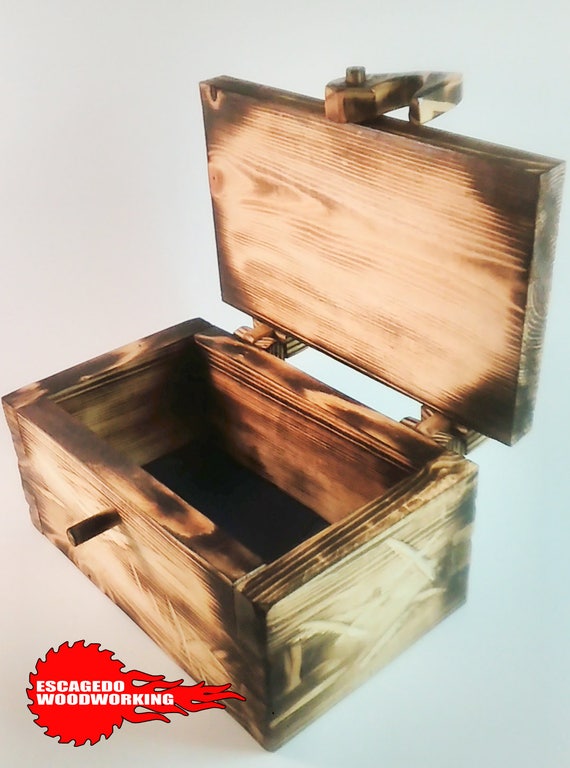The photograph features an advertisement for Escogito Woodworking, presented against a plain light gray background with hints of green on the right. Dominating the bottom portion of the image is a red outline of an electric saw, complete with a toothed gear and flames emanating from it, reminiscent of a motorcycle gas tank design. The saw prominently displays the white text, "Escogito Woodworking." The main focus of the photograph is an open wooden box, which showcases exceptional craftsmanship and a minimalist design. The box, constructed from a mix of tan and dark brown wood, exhibits wooden hinges, a wooden latch mechanism, and aged, burned edges, characteristic of a fine aging process. The interior is lined with black, contrasting the light wood exterior, and highlighting the purely wooden construction, devoid of any metal components. The attention to detail in using only wood for the hinges, handles, and latching mechanism underscores the meticulous quality and uniqueness of the woodworking on display.